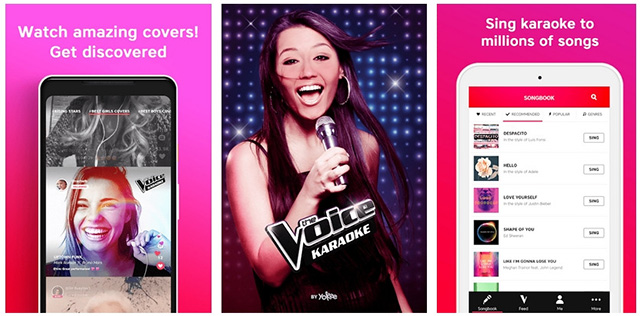This advertisement promotes the Voice Karaoke app through a visually engaging layout comprising three vertically oriented panels. 

**Left Panel:**
The left panel features a smartphone with a black bezel and silver edges against a pink gradient background transitioning from light to dark, purplish pink. The screen of the smartphone displays the Voice Karaoke app interface, showcasing a woman smiling at the screen with three indiscernible menu options at the top in white text. The selected menu option is underlined in red. Above the smartphone, white text reads, "Watch amazing covers get discovered."

**Center Panel:**
The center panel highlights the iconic logo of "The Voice" show. A young woman, approximately 18-22 years old with brunette hair and light skin, is captured mid-performance, singing into a microphone. She is dressed in a simple tank top and is standing before an LED grid backdrop emitting white lights, adding a dynamic and energetic ambiance to the scene.

**Right Panel:**
The right panel mirrors the gradient pink theme, featuring a white smartphone. Text in white reads, "Sing karaoke to millions of songs." The smartphone screen displays the app's song selection interface, complete with a red banner and search button at the top. The song list features album art thumbnails on the left and various unreadable buttons to the right, indicating the app's extensive song library.

Overall, the advertisement effectively showcases the Voice Karaoke app's engaging features and user-friendly interface, promising an enjoyable singing experience to its users.